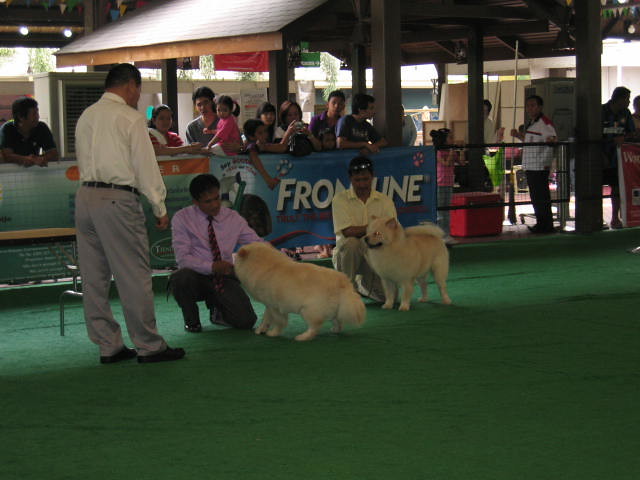This photograph captures a moment at a dog show set outdoors in the middle of the day. The foreground is covered with green artificial turf, and two fluffy, white-and-brown Pomeranian dogs are centrally positioned, being held respectfully by two men kneeling beside them. One man, dressed in a suit, and the other in a polo shirt and dress pants, are accompanied by a third man standing to their left, dressed in a shirt and tie, likely acting as a judge evaluating the dogs. Behind them is a fence adorned with banners, one prominently displaying the word "Frontline." Beyond the fence, a crowd of onlookers, mostly of Asian or Indian descent, watches intently, with a child in a pink t-shirt perched atop the fence. In the background, the setting includes some benches, a wall, various buildings, and overhead structures. The vivid colors in the image range from green and tan to white, blue, red, pink, and brown, adding to the lively atmosphere of the event.